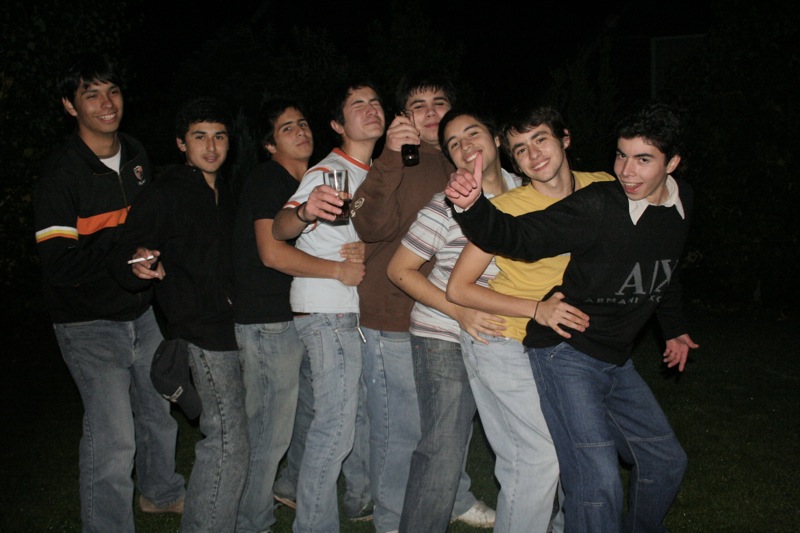In this nighttime photograph, eight young men, likely aged 18 to 24, are lined up in a conga-like pose on a dark, grassy ground. They are all adorned in various shades of blue jeans and a mix of jackets and shirts. The man at the front strikes a cheerful pose with a thumbs-up gesture, wearing a black and gray Armani Exchange sweater over a collared shirt. Behind him, a man in a yellow shirt and blue jeans smiles, holding onto the front man's hips. The third in line sports a multicolored striped polo, also gripping the hips of the person in front. The fourth individual wears a brown hoodie and holds a bottle, possibly Coca-Cola. Following him is a man with a white or light blue t-shirt accented with orange trim, closing his eyes and clutching a pint of beer. Next, a man in a black t-shirt wraps an arm around the waist of the person in front of him. The second-to-last man wears a black long-sleeve shirt and extends his right hand holding a cigarette. The final individual at the back of the line has a black jacket featuring orange and yellow stripes. All participants share smiles, adding a sense of camaraderie and fun to the scene.